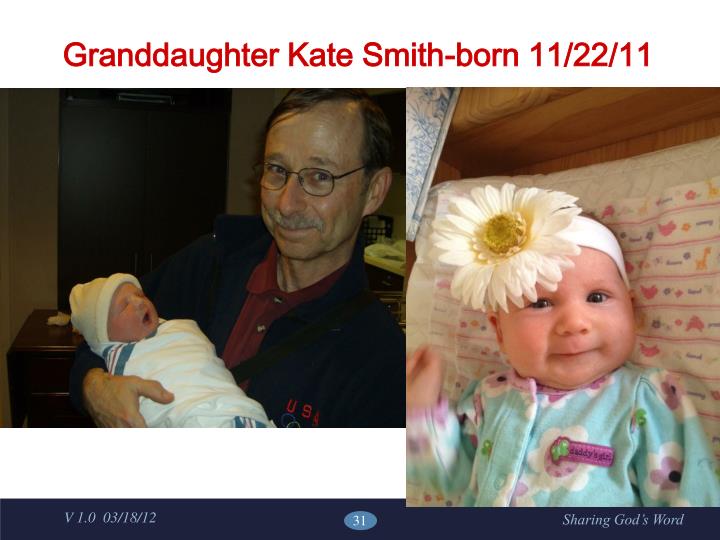The image features a white banner across the top with red text reading, "Granddaughter Kate Smith, born 11-22-11." Below the banner are two photographs side-by-side. The left photograph captures a late middle-aged white man with a receding hairline, dark brown hair, and a gray mustache. He is wearing glasses, a blue jacket over a red shirt, and holding a baby wrapped in a blue and white blanket with a stocking cap. The baby appears to be yawning, and there is a brown door in the background.

The right photograph shows the baby, now a few months old, smiling directly at the camera. She is wearing a blue and white floral onesie with purple accents and a white headband with a large daisy on it. The baby has her hand raised and is laying on a blanket featuring colorful dinosaur designs with a wooden background partially visible. Across the bottom of the frame is a blue band displaying the date 3-18-12, and in italics in the lower right corner, it reads, "Sharing God's Word."